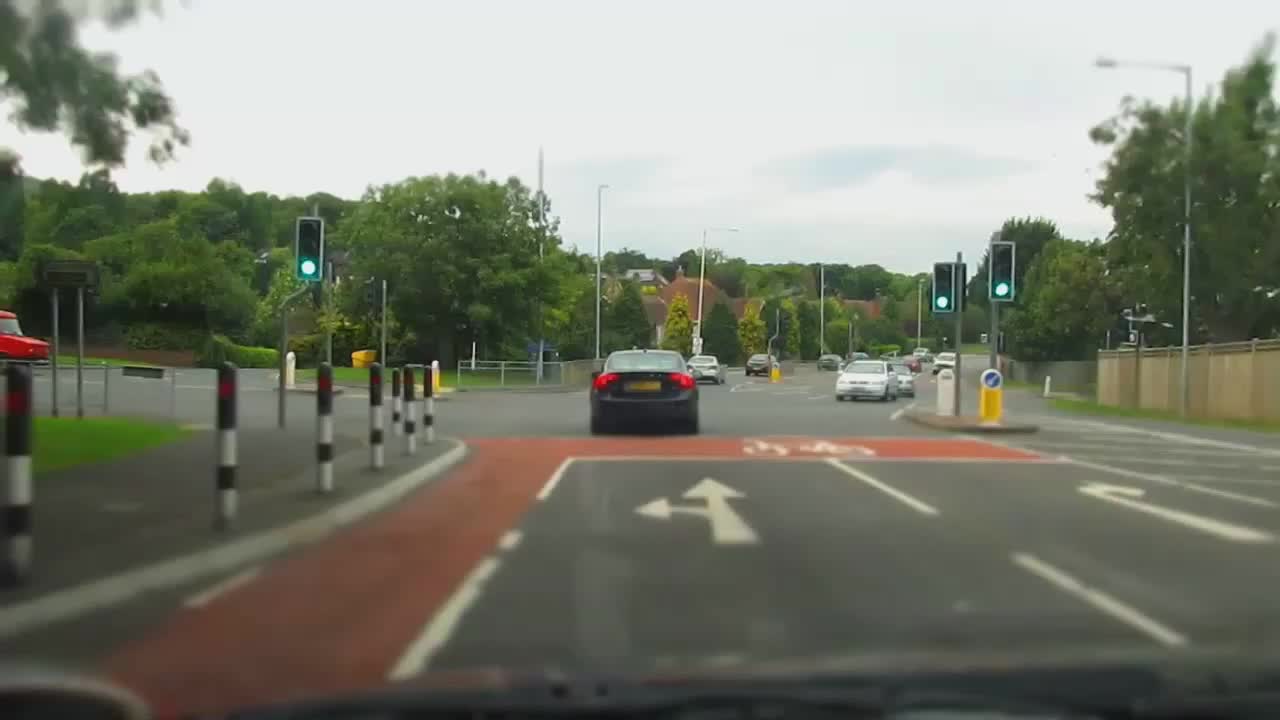The photograph captures a moment from the perspective of a driver in a black car, seemingly paused at a green light in a complex, multi-angle intersection. The road ahead includes a couple of lanes for both oncoming and ongoing traffic, with cars driving on the left side of the road, suggesting it might be situated in a country where left-hand driving is practiced. On the left side of the road are cement posts striped in black and white, possibly to delineate a protected lane or bike path, further highlighted by red brick paving, which suggests a bike lane. The intersection is marked by three green traffic signals indicating it’s clear to proceed, although the driver has stopped, allowing time to capture the scene. 

White arrows on the asphalt guide the traffic forward and to the left, while an additional arrow to the right shows a curve, contributing to the complexity of the intersection. The scene is framed by a backdrop of trees and a neatly aligned fence, adding to the organized appearance of the area. The pavement appears new and well-maintained, hinting at a location that might be somewhere like Northern California. A sense of spatial distance is inferred by the separation between the photographer's car and the next, enhancing the depth of the image. The presence of white dashed lines in the center of the road provides further directionality amid the traffic elements. Overall, the image portrays a bustling yet orderly urban roadway with clear navigational aids.